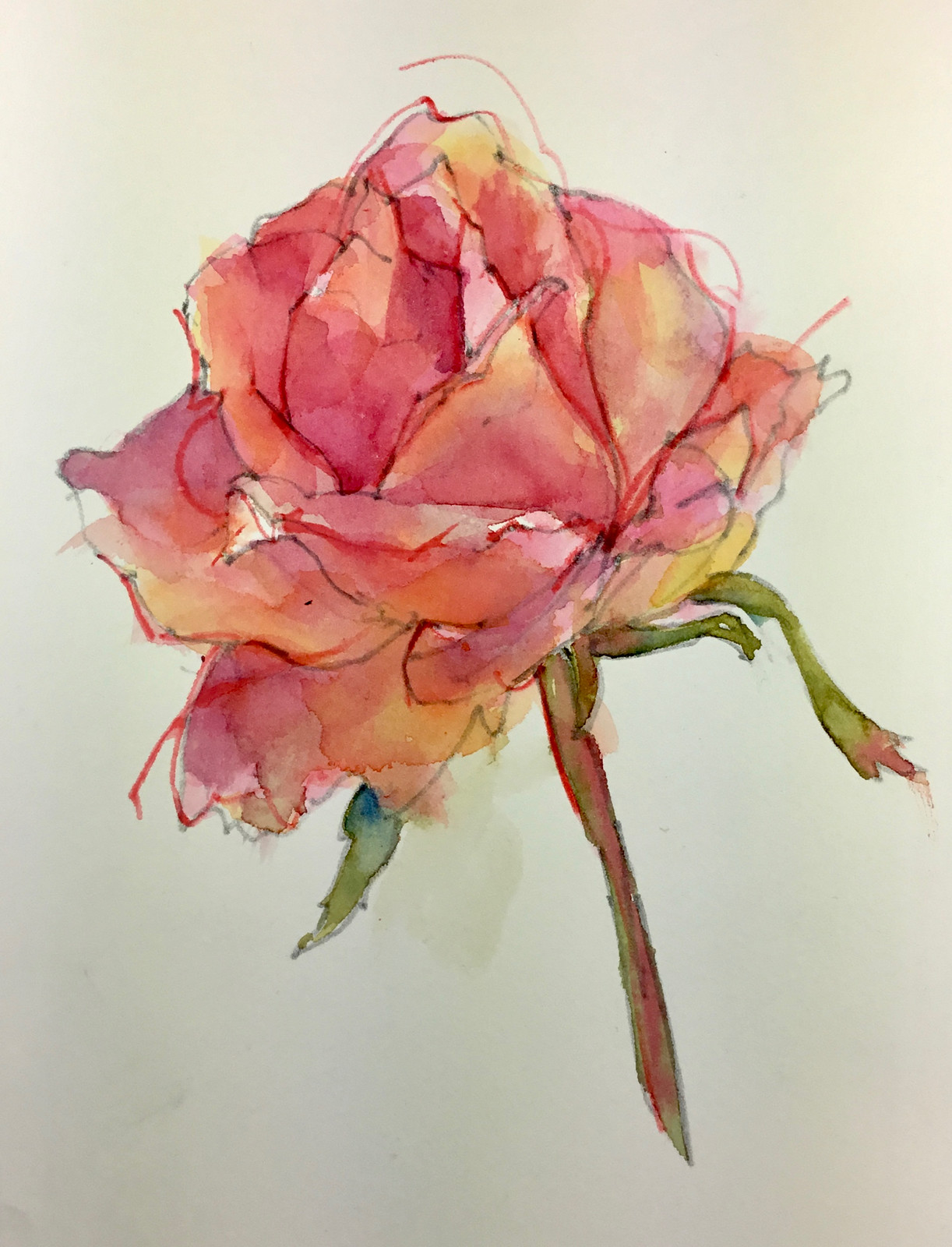This is a detailed watercolor painting of a rose blossom, showcasing a beautifully blended array of colors including peachy shades of coral, apricot, orange, yellow, red, and pink. The painting emphasizes the rose with its frayed, meticulously detailed petals that create a sense of depth and intricacy. The rose is accompanied by a green stem, which includes a small streak of red, and a few green leaves draping down from the bottom. The vibrant bloom and delicate shading bring the rose to life, set against a simple, creamy white background that accentuates its natural beauty. There are also a few wispy strings of pink extending from the rose, contributing to the distinct watercolor technique. The painting may have been initially sketched in pencil or pen, adding to the finesse of the detailed artwork.